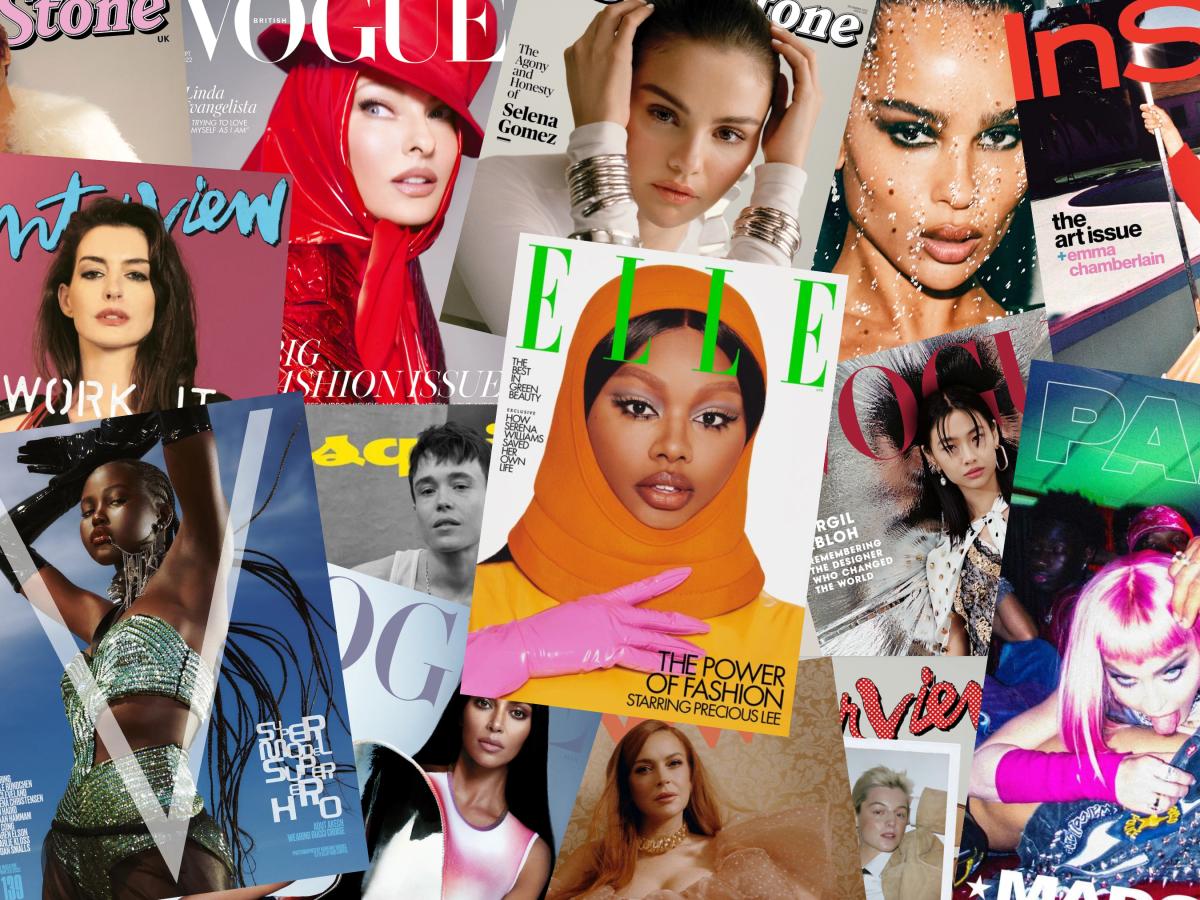This is a detailed collage of approximately 12-13 women's magazine covers, creatively overlapped in a square format. Dominating the center is an E-L-L-E magazine cover featuring Precious Lee, a black model wearing an orange hood, with the headline "The Power of Fashion." Surrounding it are various other covers, including Rolling Stone, Vogue, Interview, Esquire, and a magazine starting with P-A. These covers span a diverse array of women from different races, displaying a variety of hairstyles and fashions. Notable elements include a woman with a red hat, scarf, and coat; a bald woman in a white jacket with silver bracelets; a woman splashed with water; and another in a green top and skirt with gloves up to her elbows. Additionally, there is a unique and provocative image of a woman with pink hair licking someone's bare back in the bottom right corner. The only male presence appears to be a man with short black hair. The myriad of fonts and styles of text add to the dynamic and eclectic feel of the montage, showcasing the vast landscape of women's fashion and representation.